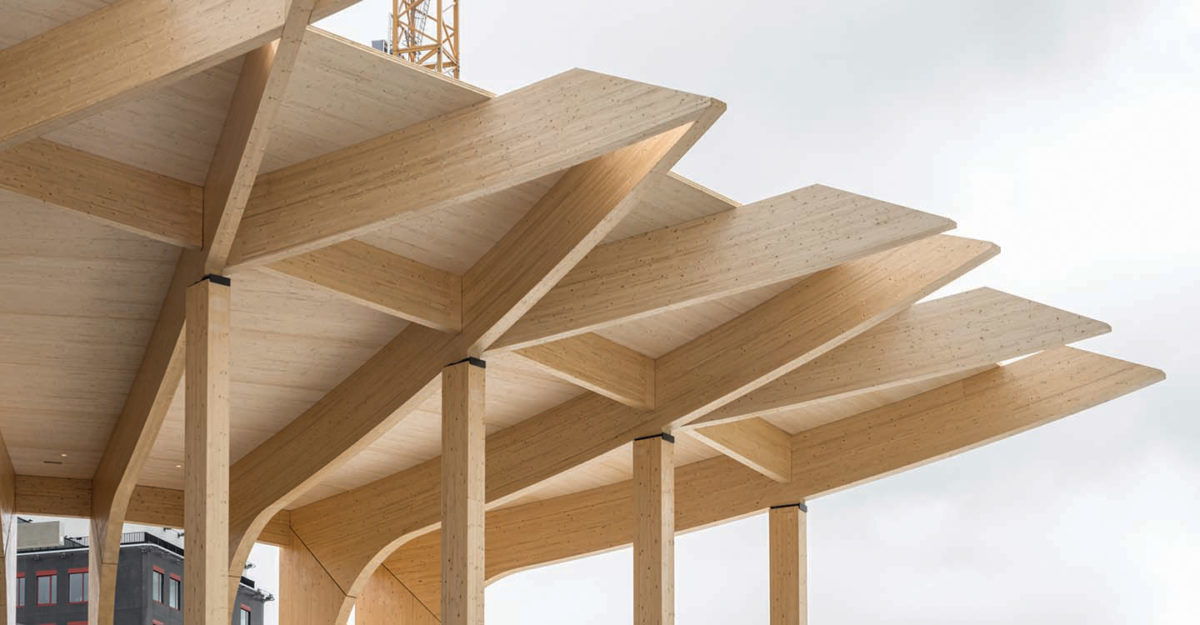The photograph captures an outdoor wooden structure that spans diagonally across the image from the upper left to nearly the right edge. The main focus is the roof-like framework, which appears to be a public structure rather than a private building. The top of the structure is composed of large, flat wooden panels, possibly plywood. These panels are supported by horizontal beams underneath and are further stabilized by diagonal and vertical wooden posts. In the background on the bottom left, there is a glimpse of a black building featuring vertical rectangular windows with red borders. The image also reveals a light gray, partly cloudy sky in the top right corner, adding to the outdoor setting. Additionally, a small metal tower is visible above the wooden structure. The predominant colors in the photo include shades of tan, yellow, red, brown, black, off-white, and gray. The photograph, taken during the daytime, highlights both the wooden construction and the modest urban environment surrounding it.